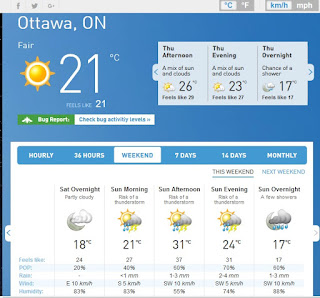Screen capture of a weather page for Ottawa, Ontario. The current weather is marked as 'fair' with a temperature of 21°C. Forecast details in Celsius indicate a high of 26°C in the afternoon, dropping to 23°C in the evening, and further reducing to 17°C overnight. Users have the option to toggle between Celsius and Fahrenheit, as well as kilometers per hour and miles per hour for wind speed measurements. The page allows sorting by hourly, 24-hour, weekend, 36-hour, 7-day, 14-day, and monthly forecasts. The weekend forecast showcases Saturday overnight at 18°C, Sunday morning at 21°C, Sunday afternoon peaking at 31°C, Sunday evening at 24°C, and Sunday overnight cooling down to 17°C. The date is not displayed, making it unclear whether this is a spring or fall forecast.